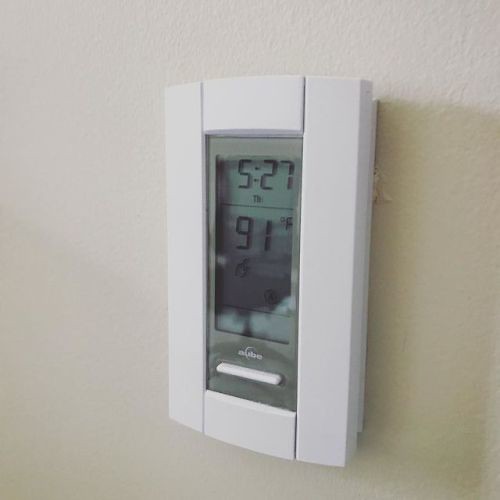A digital device with a white plastic casing is mounted on a slightly rough, white-painted wall. The LCD display at the top shows the time "5:27," while below it, the temperature is displayed in degrees Fahrenheit as "91." The black numbers are clearly visible against the screen, which has a slightly greenish tint. At the bottom of the display, there is a thin, white, elongated button. The device appears to be affixed to the wall using double-sided sticky foam, some of which is visibly protruding from behind the white plastic casing.